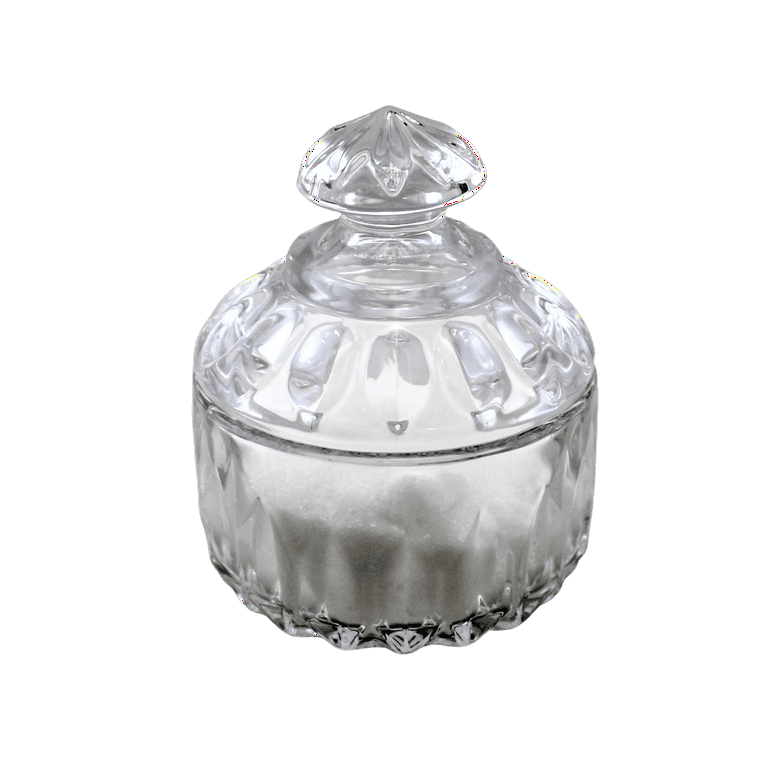The image depicts a round, cup-shaped jewelry container or sugar jar, floating against a white background without any borders or additional imagery. The main body of the container is relatively plain and cylindrical, made of clear glass with a slightly meadow-like appearance. The container is filled with a crystal-like substance, possibly sugar or salt. 

The lid is highly decorative and constitutes about one-third of the overall height. It's adorned with squarish, refractive glass pieces embedded along its edge, creating a shimmering effect. At the top, the lid tapers into a dome that features similar glass pieces, continuing up to a small, pointed handle or knob at the top, which also has intricate engravings resembling thumb-sized bumps and additional embedded glass pieces. The knob has faint, white lines with tiny red-yellow dots, adding to its antique aesthetic. The metal elements at the bottom of the container also have some ornate design, with glass pieces attached to the corners, providing a touch of elegance and shine.

Overall, the container has an antique feel, with detailed engravings and embedded glass elements enhancing its decorative appeal.